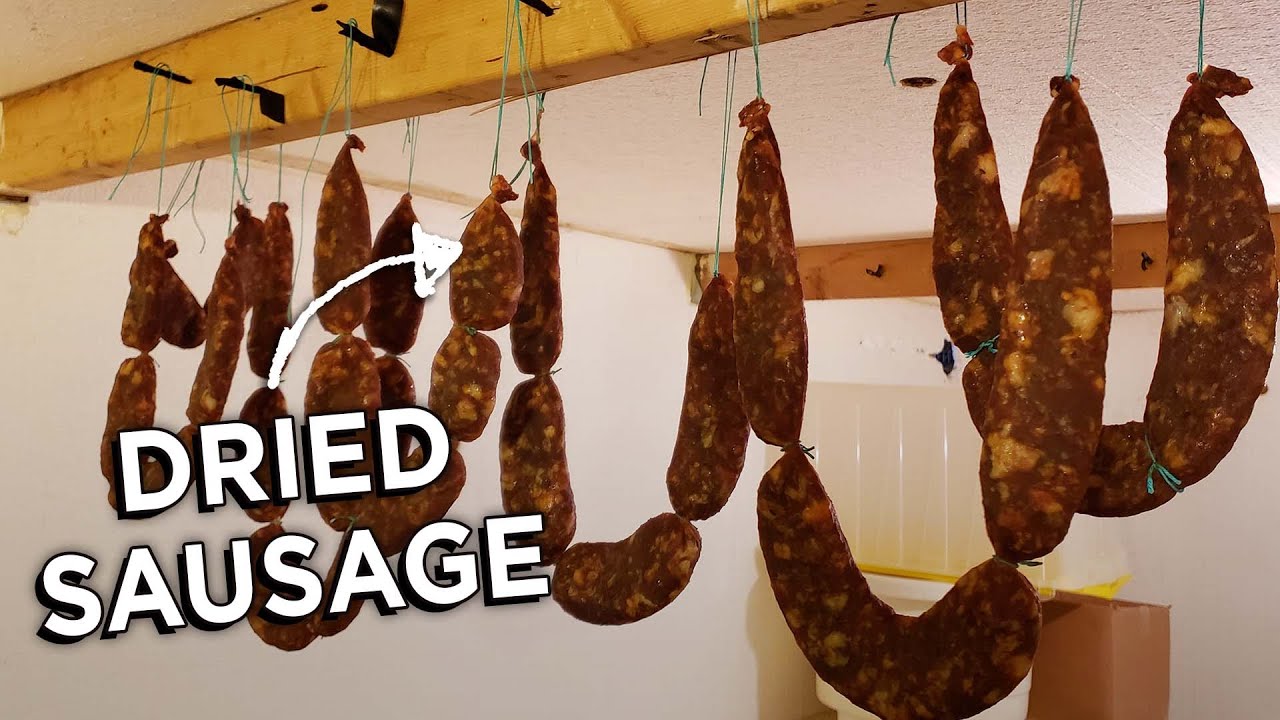The photograph depicts a collection of brown dried sausage links hanging in various u-shapes from the ceiling. These sausages, strung together with thin green cords, dangle from screws embedded in wooden runners or beams that appear yellow in the image. Each screw is connected to black hooks which securely hold the sausages in place. There are six or seven sets of sausage links, each set containing three to four thick sausages with visible white fat pockets. A white text overlay with the words "dried sausage," accompanied by a scribbled white arrow, points towards the sausages. The room, potentially a kitchen, has a white interior, though specific details of the surroundings are obscured by the prominence of the hanging sausages.